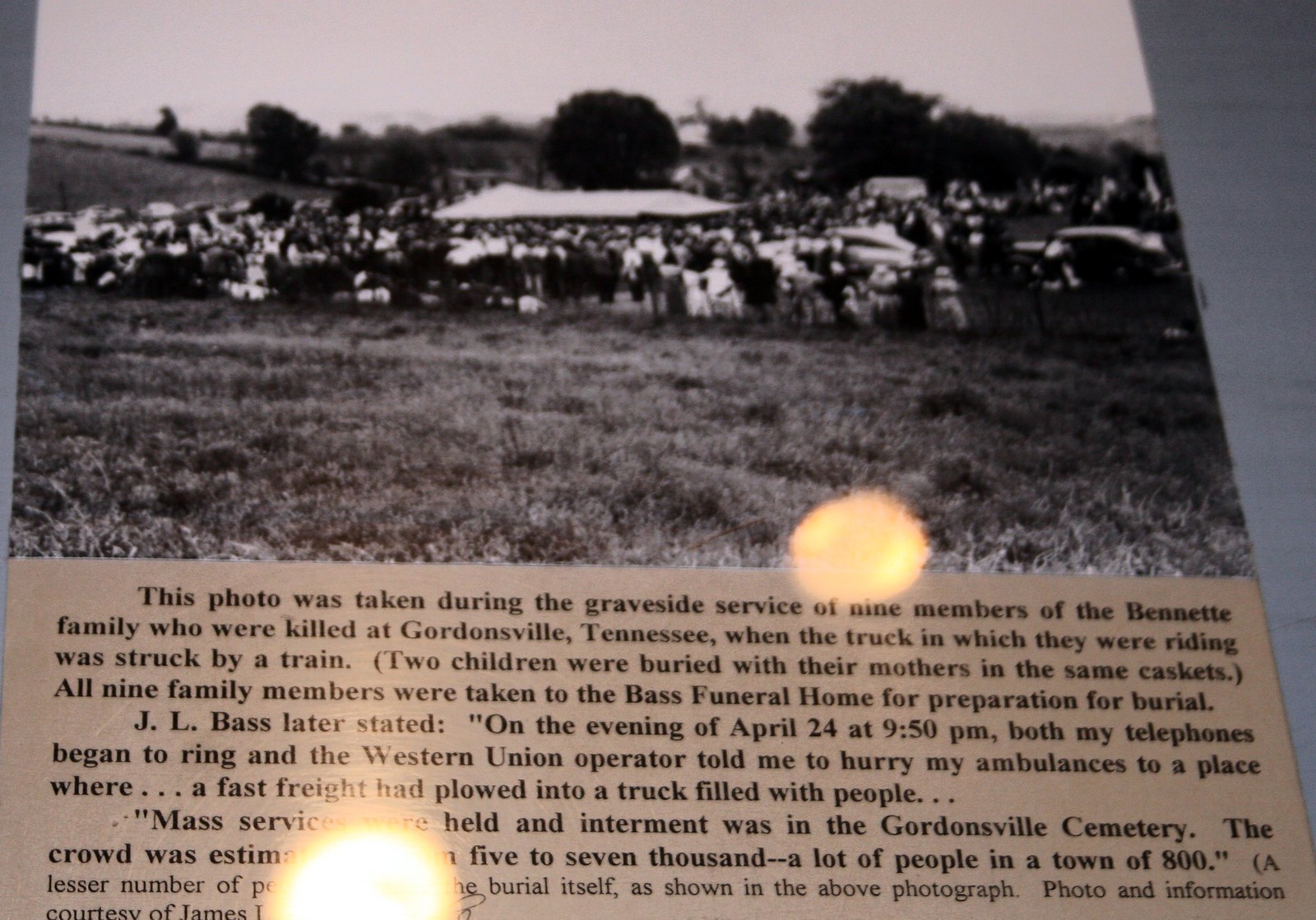This is a blurry black and white photograph, likely taken from a magazine or old newspaper, showing a large crowd gathered in an open field for a somber occasion. The backdrop includes some distant trees under a gray, cloudy sky, with a white tent canopy central to the scene. The event captured in this image is the graveside service for nine members of the Bennett family, who tragically perished in Gordonsville, Tennessee when the truck they were riding in was struck by a train. All nine victims were prepared for burial by Bass Funeral Home, and the mass service drew an estimated crowd of 5,000 to 7,000 people, a significant turnout for a town of just 800 residents. Notable in the description is that two children were buried with their mothers in the same caskets. J.O. Bass, from Bass Funeral Home, recounted receiving an urgent call from the Western Union operator on the evening of April 24th at 9:50 p.m. about the swift freight train disaster. The photograph captures a quieter moment of the ceremony, contrasting with the massive attendance estimated overall.